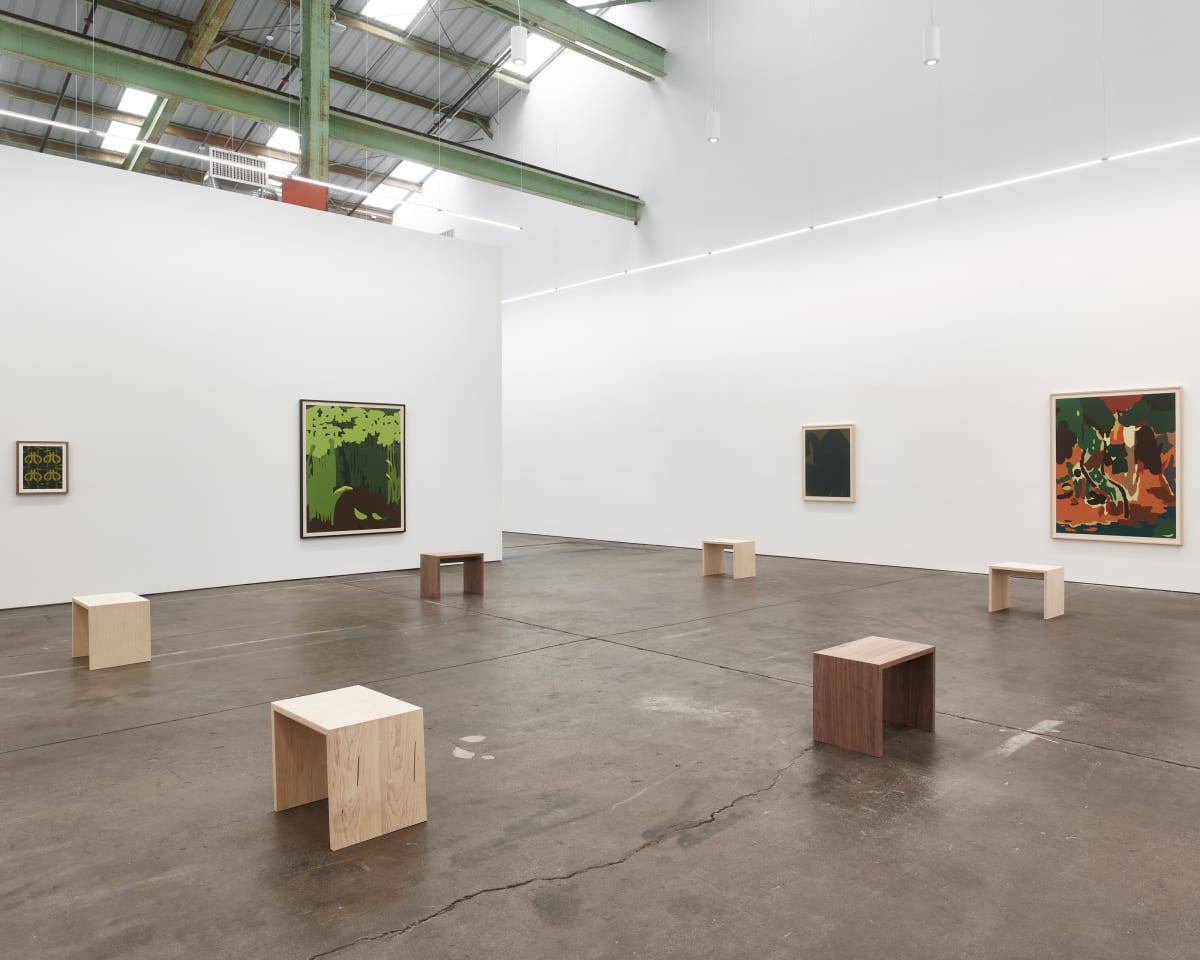The photograph captures an art gallery with white walls and an unfinished, corrugated metal roof featuring rectangular skylights that allow natural light to filter in. Green-painted steel support beams and pillars are visible in the top left corner. The unfinished concrete flooring is partially covered with slabs, one of which, near the bottom center, is cracked. Arranged in a circle on the floor are several small, three-sided wooden chairs; some are made of light white-colored wood and others of darker-colored wood. Four abstract paintings in various square frames are displayed on the white walls: the smallest on the left, a larger one towards the center, another small one that appears black a bit more to the center right, and the largest on the far right. The image, taken in landscape orientation, employs artificial light but also makes use of natural light from the skylights, creating a detailed, realistic depiction of the space.